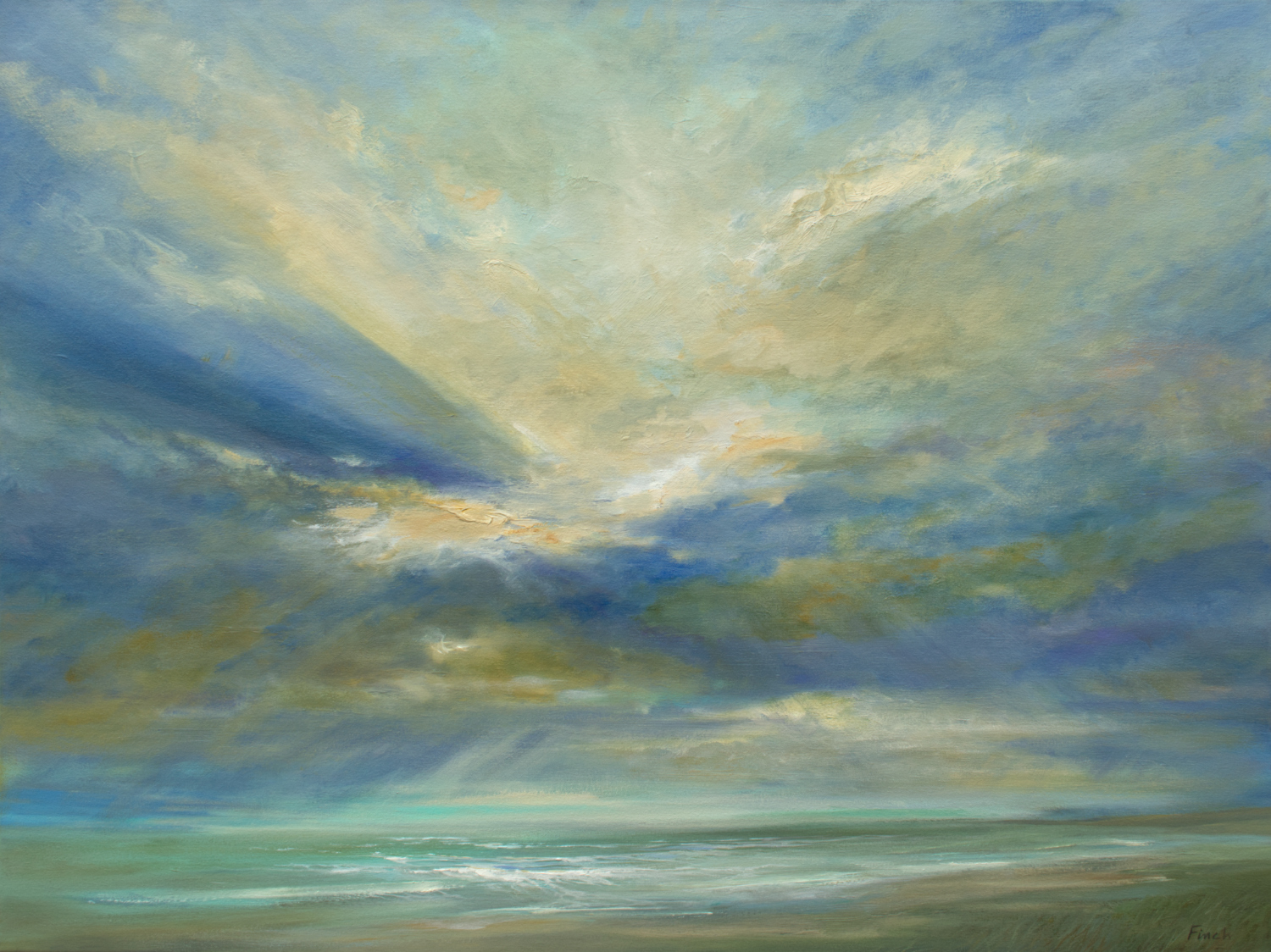The painting, rendered in either aureole or acrylic paints, portrays an abstract yet vivid sky at either sunrise or sunset. Dominated by a gradient of blue and yellow hues, the sky exhibits a spectrum of colors that move from white and yellow at the center—suggesting the sun's radiant position—to darker blues and purples, with hints of green and yellow in the clouds below. Sunbeams subtly penetrate through the clouds, adding to the ethereal quality of the scene. Beneath the sky, the painting transitions into a turquoise strip of water, seamlessly blending into the horizon where the sky meets the sea. The presence of white waves crashing onto a sandy beach on the right-hand side further enhances the tranquil, natural setting. The overall composition, minimalistic and shape-free, elegantly captures the harmonious confluence of sky and sea in a distant, serene vista.